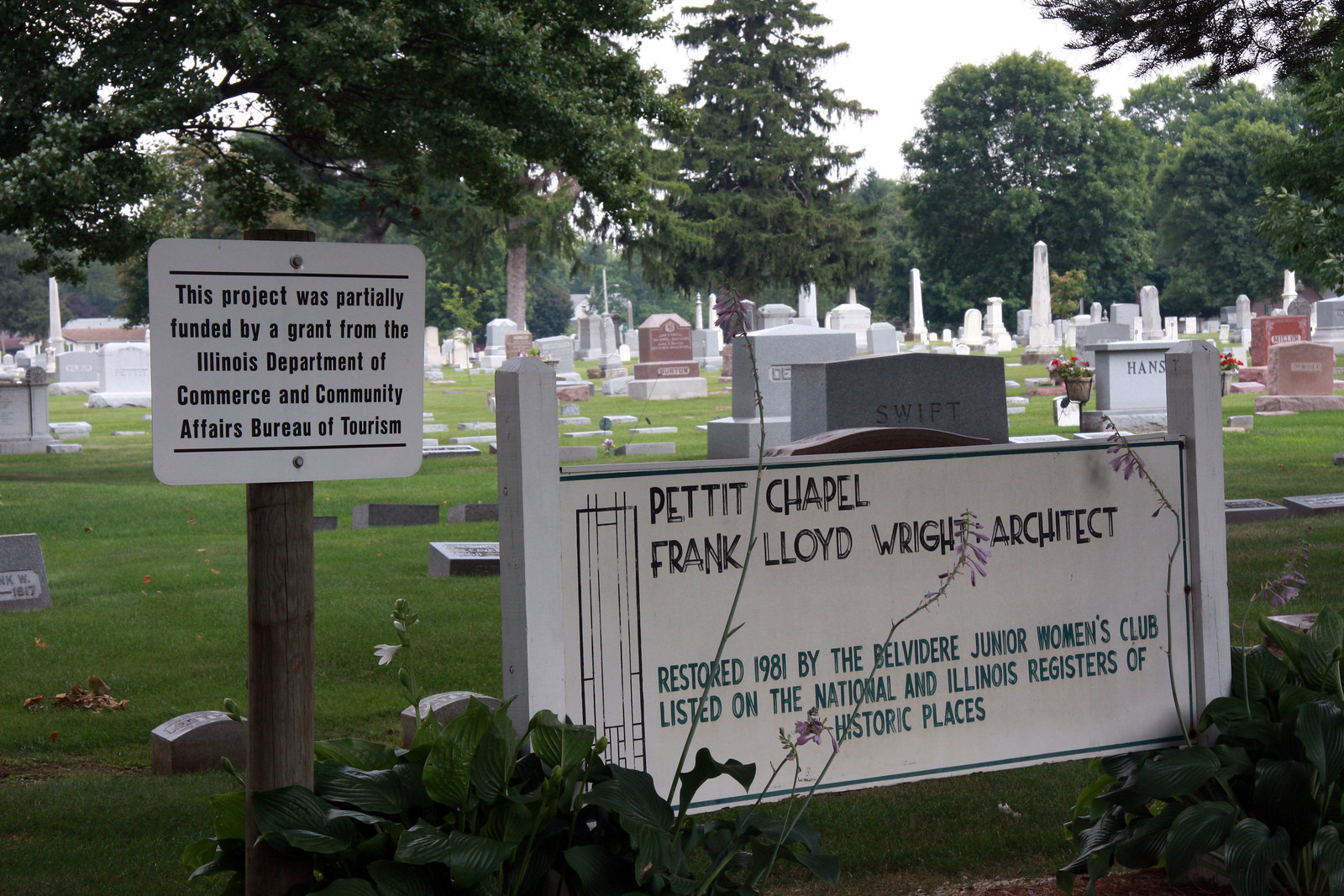The image depicts a sprawling cemetery bathed in greenery, with lush grass carpeting the ground. Tall trees are scattered throughout the background, creating a serene yet slightly shaded ambiance in the front section. The sky above is a clear and uniform white, enhancing the tranquil atmosphere. Among the greenery, various tombstones of differing sizes and colors—primarily white, gray, and some reddish stones—stand in poignant contrast to the vibrant grass.

On the left side of the image, there is a wooden post bearing a sign that reads, "This project was partially funded by a grant from the Illinois Department of Commerce and Community Affairs Bureau of Tourism." To the right, a more prominent white wooden sign stands, inscribed in black letters with the details: "Petit Chapel, Frank Lloyd Wright Architect, Restored 1981 by Belvedere Junior Women's Club, Listed on the National and Illinois Registers of Historic Places."

This detailed scene captures the essence of a historically significant and meticulously maintained cemetery, with the notable architectural contribution of Frank Lloyd Wright highlighted amidst the resting stones.